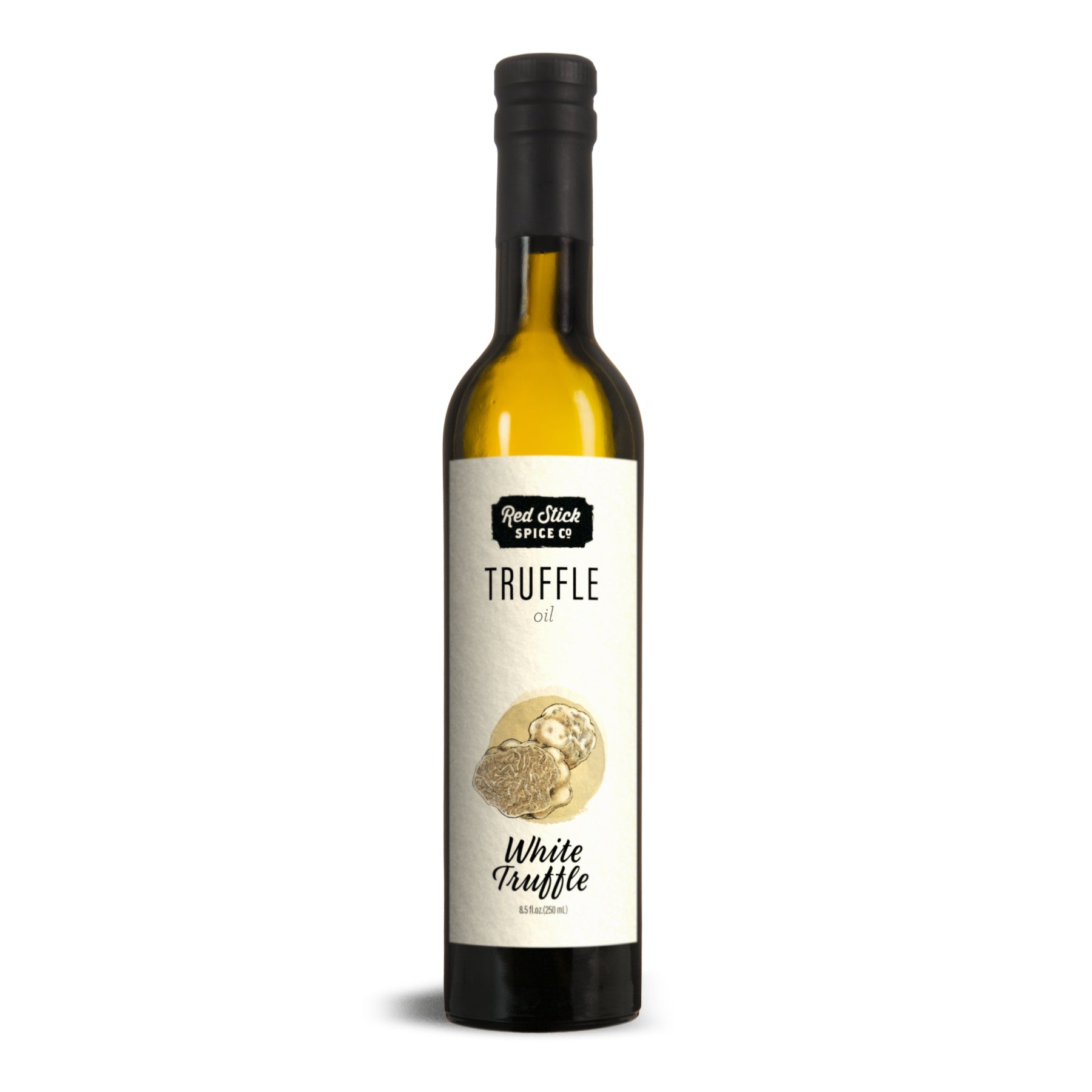This image features a long, thin bottle of white truffle oil from the Red Stick Spice Company. The bottle is tinted yellowish and darkens towards the bottom, almost to black, giving it an amber-green appearance. It stands upright, with a slight shadow cast to the left. The bottle is sealed with a black cap and has black wrapping around the lid. The label is a simple white sticker with black text. The brand name, "Red Stick Spice Company," is highlighted in white on a black rectangle. Below the brand name, "white truffle" is printed, along with an illustration of a truffle, which resembles either a cauliflower or a mushroom. The contents of the bottle appear yellowish but are much darker at the bottom, indicating settling of the oil.